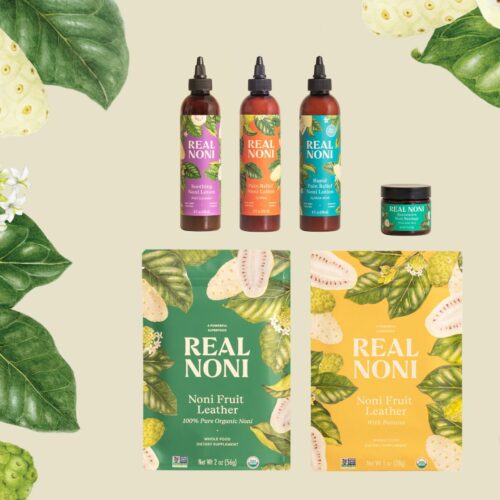The image is a commercial product photograph featuring a lineup of items from the brand "Real Noni" against a creamy white background. The background is adorned with leaves, flowers, and fruit from the Noni plant native to Hawaii, creating a natural, organic ambiance. On the left side of the image, lush green leaves and vibrant fruit clusters contrast with the sophisticated display of products. Near the upper right corner, three bottles with black squeeze tops stand tall, labeled with large white text reading "Real Noni." Each bottle features a distinct label color: purple, orange, and blue, indicating different scents or formulations of restorative lotion and pain relief. Below these, a small glass jar with a black lid, labeled "Real Noni" in white text and adorned with a light green label, contains restorative Noni bandage with aloe vera. At the bottom of the image, two pouches showcasing different flavors of Noni fruit leather boast the claim "100% pure organic Noni." The packaging throughout the photograph varies in color, including yellow, purple, orange, aqua, and mint green tones, creating a vibrant and appealing visual presentation.